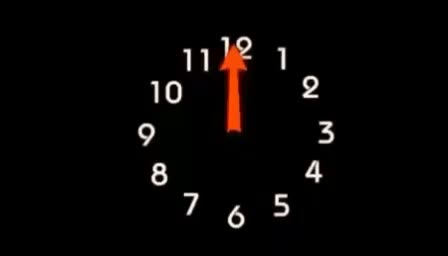This image showcases a minimalist clock featuring no casing, presenting an uncluttered, stark design. The clock face features white numerals indicating the hours from 1 to 12, distinctly displayed against a black backdrop. Notably absent are any markers for seconds, focusing purely on the main time indicators. The clock's hands, including the hour, minute, and second hands, are all prominently highlighted in red. The hour and minute hands are slender and extend prominently across the clock face, enhancing readability. Particularly, the long, arrow-tipped hand seen in the image stretches from the central axis outwards and overlaps the numeral 12, positioned between the 9 and 3 o'clock markers. This bold contrast of red and white on black creates a striking visual, emphasizing both function and modern aesthetics.